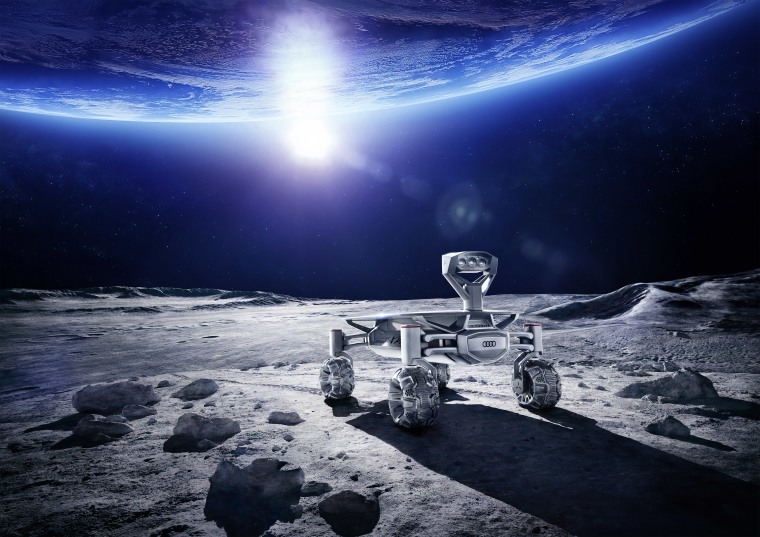The image portrays a slightly rectangular, almost square-shaped frame featuring a small rover-type vehicle on a barren, rocky, gray landscape, resembling the moon. This compact vehicle has four small, rugged tires and a flat, rectangular body with chrome-gray coloring. Mounted on top is a robotic head or sensor device, possibly for cameras or data collection, casting a shadow behind it. Directly above and dominating the upper part of the image is a large, curved section of Earth, presenting a striking blue and white pattern against the dark backdrop of space. Just below Earth appears a bright white celestial body, likely the Sun, emitting a glow that adds a vivid contrast to the scene. The surface of the moon around the rover is characterized by a blend of smooth areas and scattered rocks, particularly noticeable in the lower left corner. The meticulous details and the overall composition suggest that this image could be the work of a highly skilled graphic artist, evoking a science-fiction atmosphere.